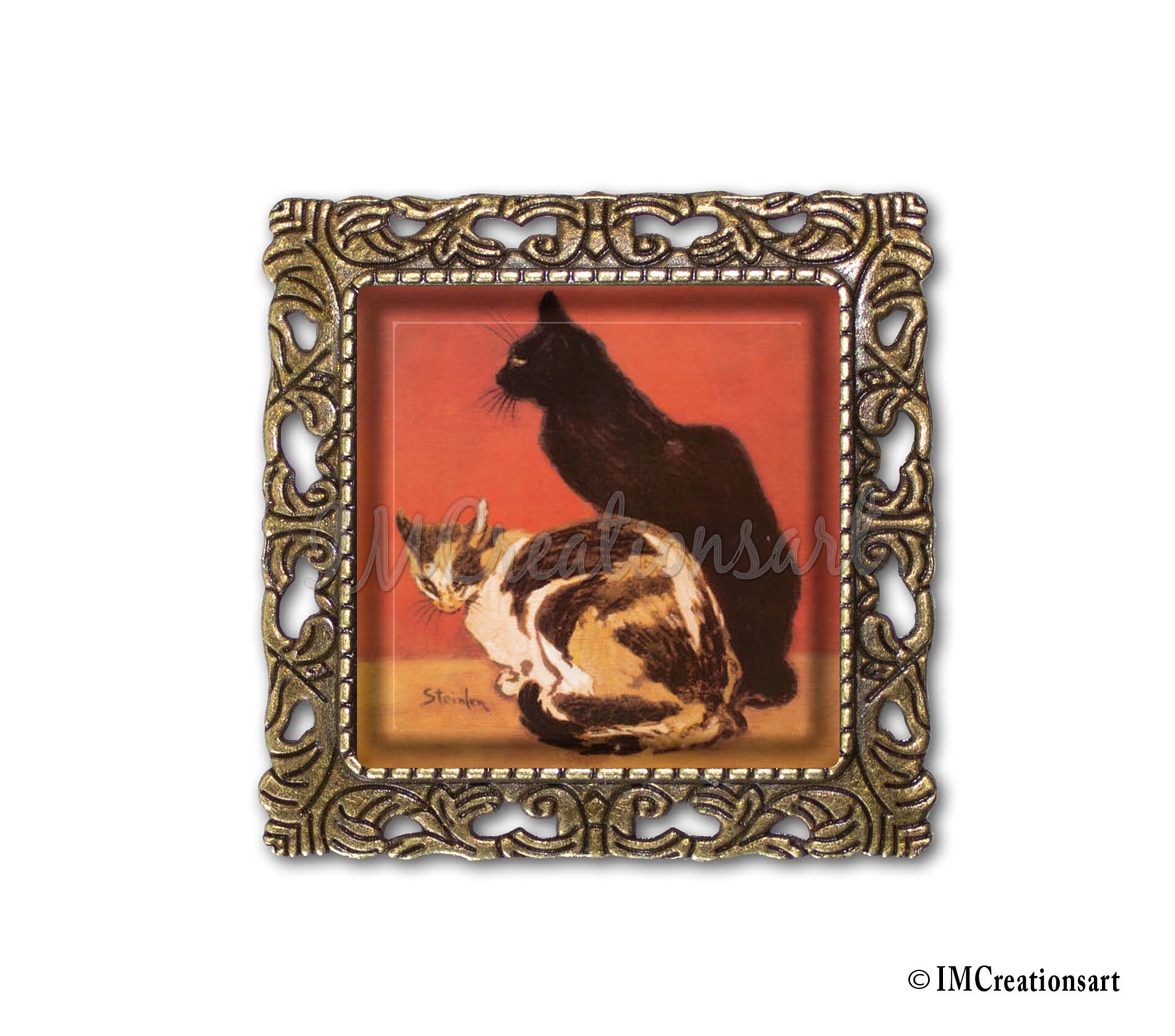This image showcases an intricately framed square painting mounted on a white wall. The frame is brass-like with a detailed, leafy design that adds an elegant touch. The painting features two cats situated against a vivid red backdrop, with an orange floor grounding the scene. The cat in the foreground, depicted in a mix of white, brown, orange, and black hues, is sitting and facing the viewer. Its posture suggests a relaxed yet contemplative mood. Behind it, a pitch-black cat is seated, gazing to the left. Notably, the artwork bears the signature "Steinlein" on the bottom left and a watermark from "I Am Creations Art" on the bottom right, both inscribed in black. The painting captures a serene moment, expertly blending color and composition to draw viewers into the tranquil tableau.